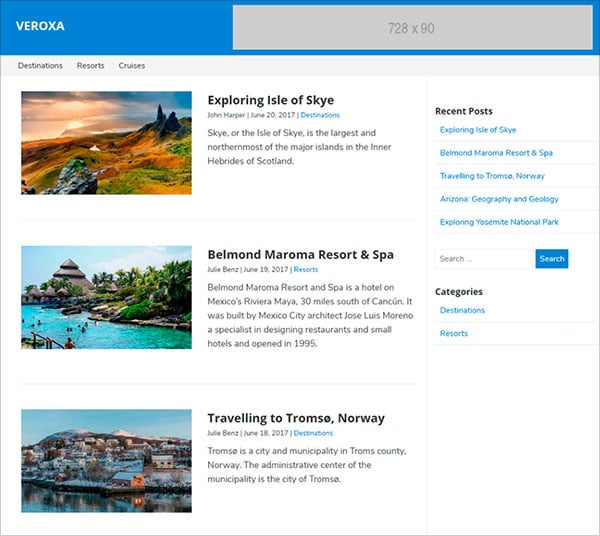Veroxa is prominently displayed in white text against a blue background. Adjacent to this, slightly grayed out, is the dimension specification "728 x 90," which appears to indicate the dimensions of this section. Below Veroxa, aligned to the left, are categories labeled as Destinations, Resorts, and Cruises. Each category features an image and text description.

The first image showcases a stunning sunset over a rugged mountain terrain, promoting an article titled "Exploring the Isle of Skye." It includes the author's name, the date of publication, and a brief introduction stating that the Isle of Skye is the largest and northernmost of the major islands.

Next, there is an image of a luxurious pool area framed by palm trees with a pyramid-shaped structure visible in the background. This image accompanies an article about the "Belmont Moroa Resort and Spa," located 30 miles south of Cancun. The author and date are noted, along with a snippet describing the resort.

The third image features a picturesque waterfront in Tromso, Norway, characterized by closely-knit houses scattered along a hillside under clear blue skies. This visual ties into an article on traveling to Tromso, Norway, complete with the author’s name, date, and a brief summary.

To the right, a bold header titled "Recent Posts" lists articles including "Exploring Isle of Skye," "Belmont Moroa Resort," among three others, all in blue. Below this, a search function is provided with a clickable search button. The section concludes with a "Categories" list, highlighting "Destination Resorts" in blue text.